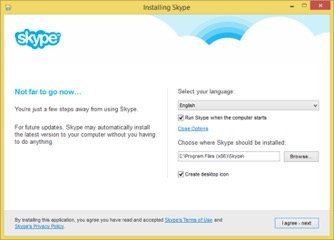The image depicts a small, low-quality screenshot of a pop-up menu related to the installation of Skype. The pop-up is bordered by a mustard yellow frame, with the text "Installing Skype" in gray font at the very top. In the upper right corner of this mustard yellow border, there are three icons: minimize, maximize, and close (X).

The menu itself has a white background. In the upper right corner, there is a blue rainbow graphic, while in the upper left corner, the Skype icon is displayed. The Skype icon consists of the word "Skype" in white font with a blue outline.

Below the icon, the text "Not far to go now..." is displayed in blue font, and underneath it, in black font, is a message that reads: "You're just a few steps away from using Skype. For more updates Skype may automatically install the latest version to your computer without having to do anything."

To the right of this message, there is an option to select your language, with English being the selected language. Below this, a checkbox is filled next to the option "Run Skype when the computer starts." Further down, there is blue font text that says "Clear cache," followed by another option to choose where Skype should be installed.